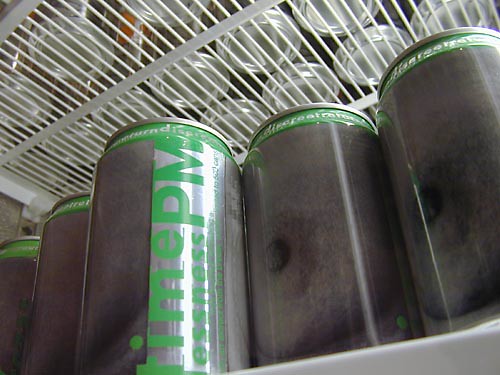This detailed color photo captures a drink fridge stocked with numerous aluminum cans. The fridge features white wire shelving, and the bottom of the top shelf is visible. The main focus is on a row of gray canned beverages, each with a green trim and green writing. The cans appear to have a partially obscured logo that reads something like "Prime PM" or "Lime PM," followed by an ambiguous word that might be "Essences." Shadows cast over the cans provide depth, enhancing the realistic feel of the image. There are at least five cans prominently in the foreground, and more cans are visible on the shelf above, making it look like there could be about a dozen or more in total.